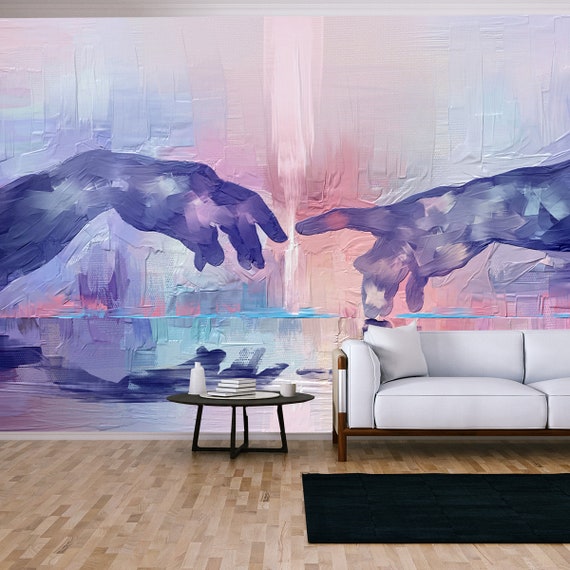In this indoor photograph of a living room, the hardwood floor is composed of small wooden pieces, and a black modern rug partially covers it. The focal point of the room is a white upholstered couch with a low back, substantial cushions, and a wooden frame, positioned slightly to the right. Adjacent to the couch is a sleek black coffee table featuring a modern design, with about five books, a coffee cup, and various small canisters arranged on its surface. The left side of the couch is accompanied by a small round side table adorned with ceramic knick-knacks. Dominating the background is a large mural, reminiscent of Michelangelo's ‘The Creation of Adam,’ depicting two hands nearly touching with a vibrant burst of lightning between them. The mural is an abstract composition filled with swirling shades of purples, blues, and pinks, enveloping the room in a dynamic and artistic ambiance. This intricate and vivid wall art draws significant attention, contrasting elegantly with the room's modern and sophisticated decor.